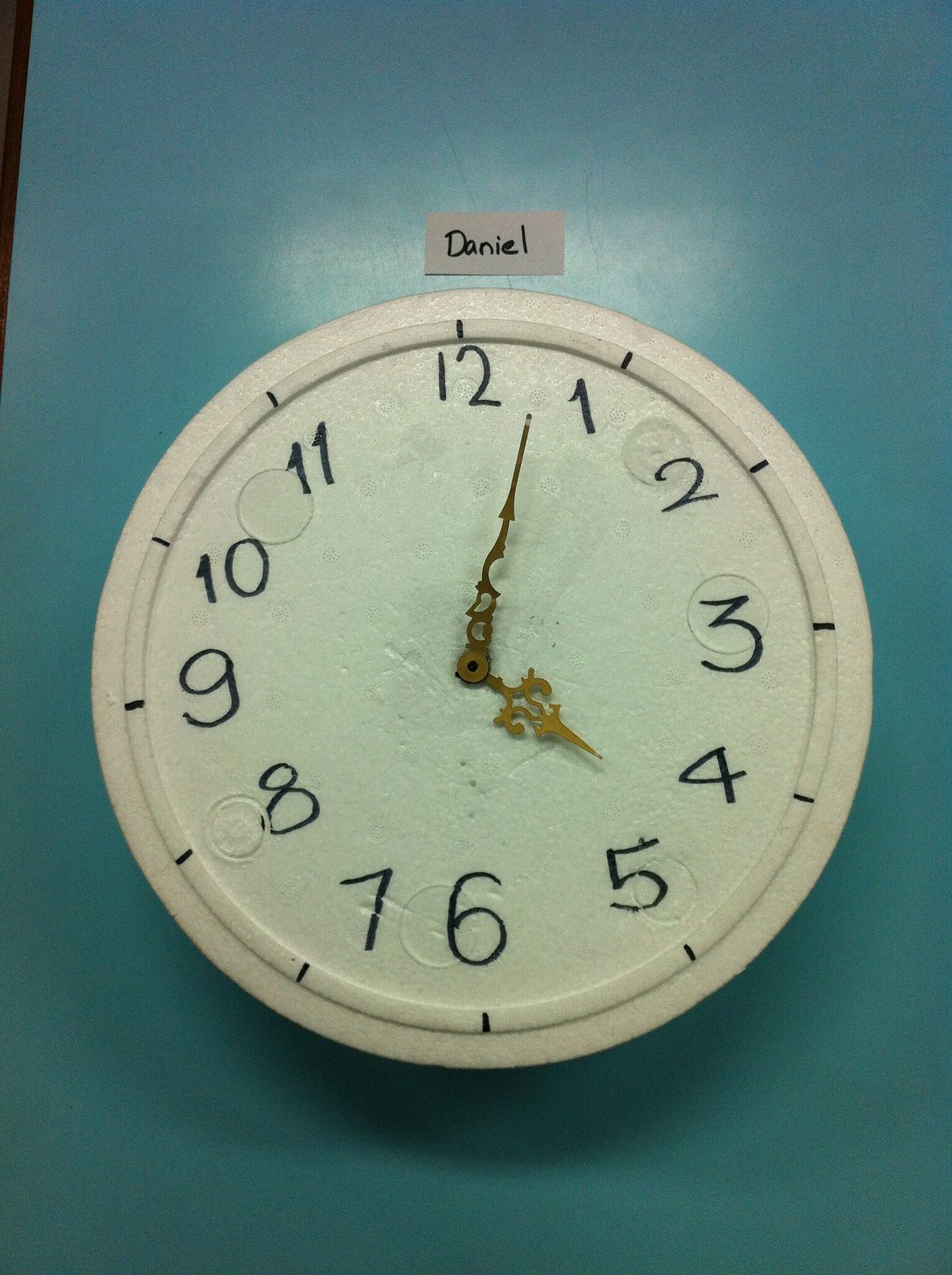This image features a homemade clock crafted from styrofoam. The clock's structure appears to include intricately designed components with the hour and minute hands resembling gold in color and material. The time displayed on the clock reads approximately 4:02. This unique, handcrafted timepiece showcases creativity and resourcefulness in its design.